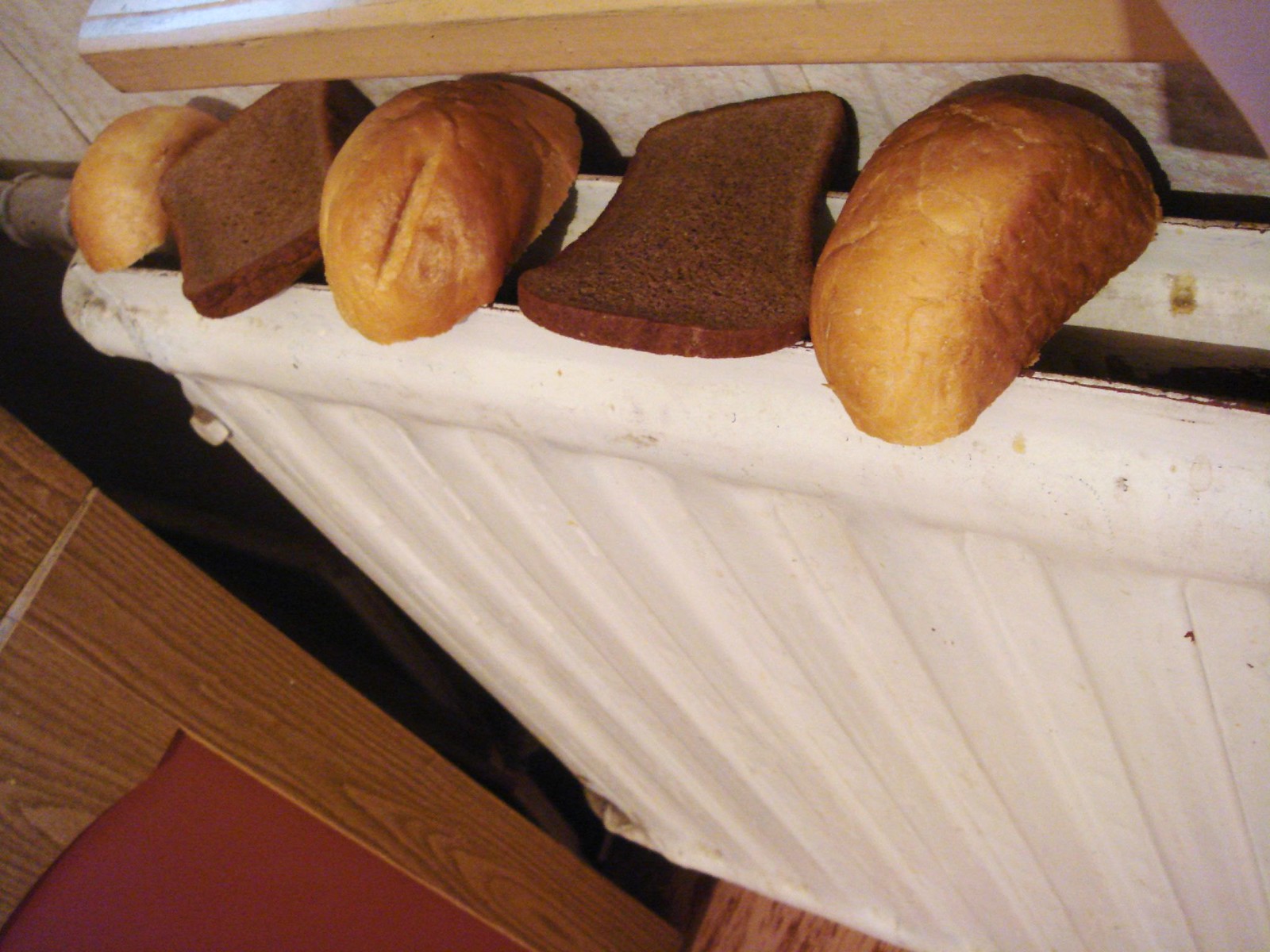This photograph, taken from an elevated perspective, features five pieces of bread resting on what appears to be an old, white-painted floor radiator, likely vintage given its slightly worn and discolored surface. The radiator heater, positioned beneath a beige windowsill, has a central open area framed by two long, rectangular heating strips, and a visible piping section. The bread pieces are arranged in a distinctive alternating pattern: three golden-brown French rolls or loaves cut in half, interspersed with two slices of dark brown rye or pumpernickel bread. This arrangement creates a sequential pattern from left to right: roll, dark bread slice, roll, dark bread slice, and roll. Around the radiator, elements of the room are faintly visible, including a brown wooden floor, wood paneling or furniture to the left, and a hint of a maroon-colored cupboard. The overall setting has an aged but homey feel, emphasized by the wooden textures and the radiator's old-fashioned design.